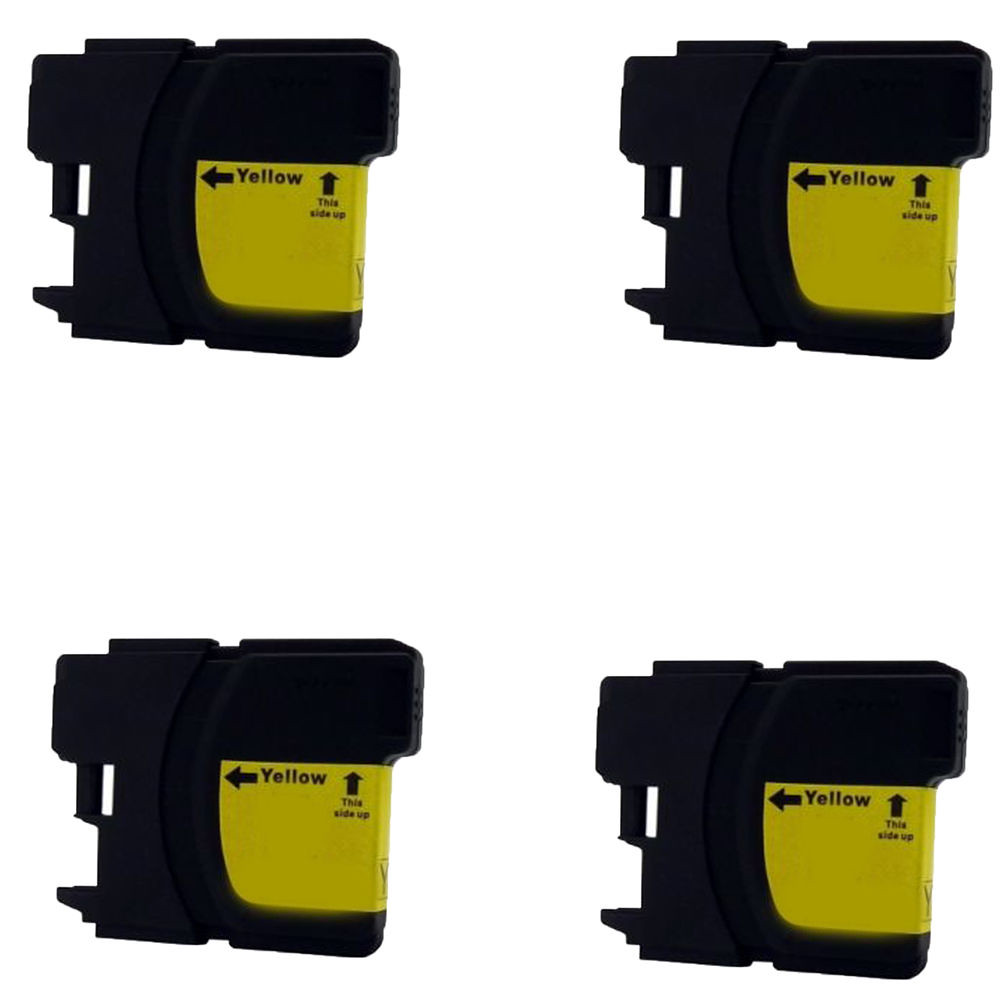The image features four identical black box-like objects arranged in a square formation on a white background, with two objects on the top row and two on the bottom. Each object appears to have a handle-like groove and prominently displays a yellow strip on the right side, which covers approximately one-quarter of the entire object. This yellow section contains black text reading "Yellow" with a black arrow pointing left, and another arrow indicating "This Side Up" pointing upwards. The yellow strip seemingly wraps around to the unseen back side of each object.